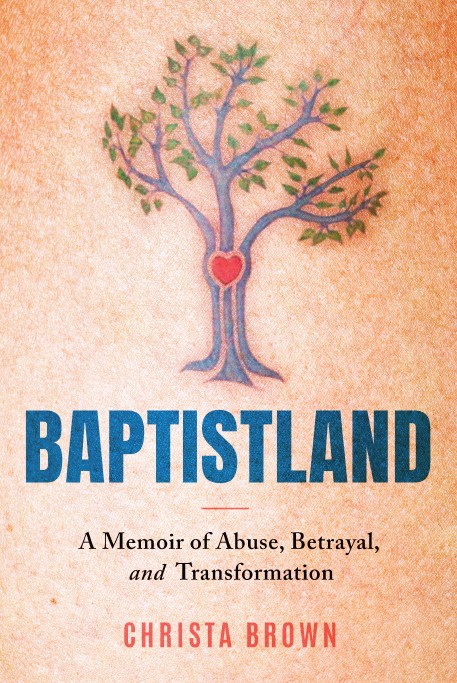This book cover features a textured light orange background that transitions to a darker orange at the top left, top right, and bottom right corners. Prominently displayed in the middle is an illustration of a tree with a singular trunk that branches into three main segments, forming a blueish hue. Nestled in the center of these branches is a distinct red heart. The tree also has scattered green leaves, adding a touch of natural detail. Below the tree, the title "Baptist Land" is boldly printed in dark blue text. Beneath the title, the subtitle "A Memoir of Abuse, Betrayal, and Transformation" is presented in black text. At the very bottom of the cover, the author's name, Krista Brown, is prominently displayed in red.